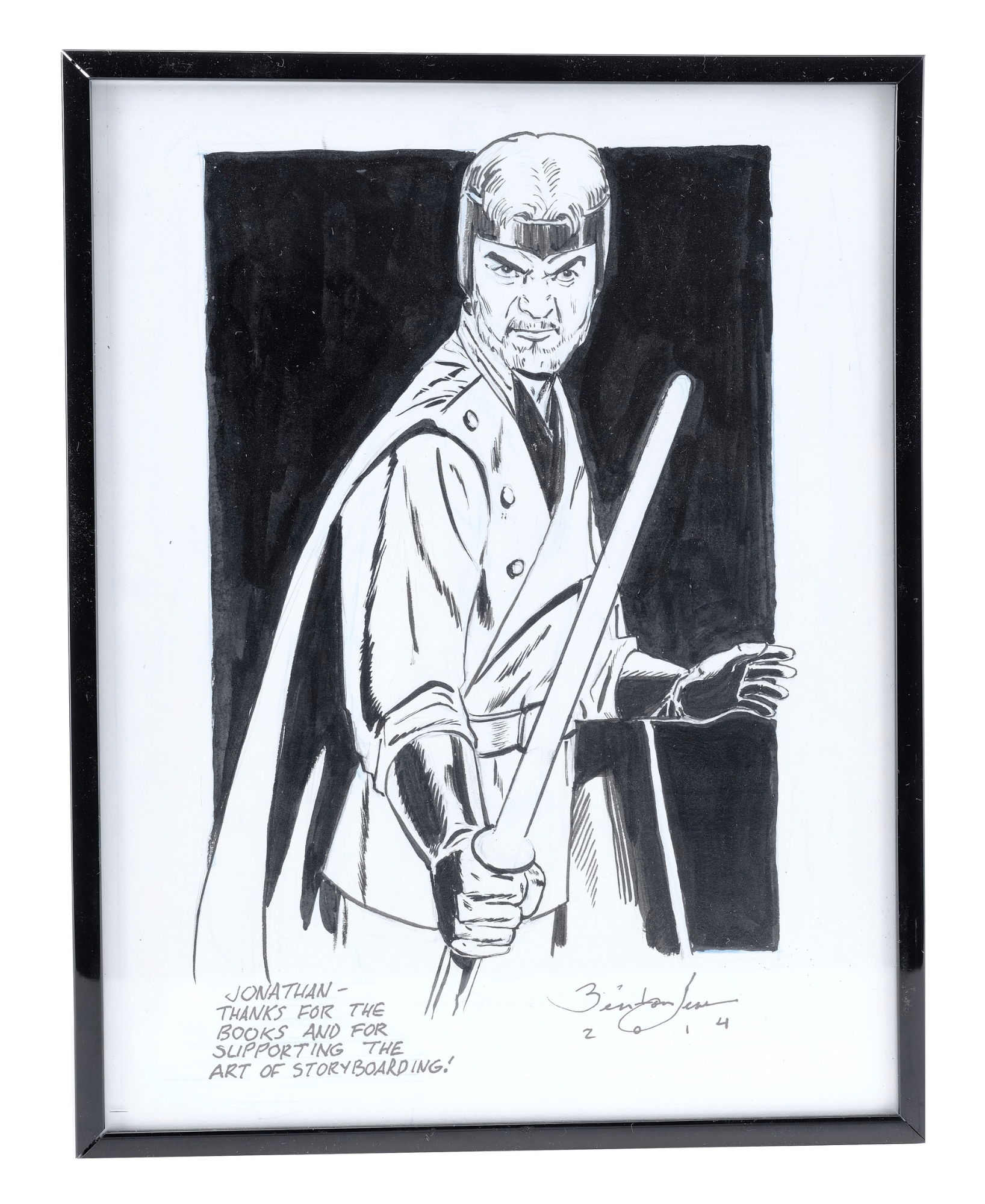This black and white hand-drawn art piece, set in a black picture frame, depicts a character resembling the late actor Sean Connery. The character is portrayed with a headband, a cape, and gloves, holding a lightsaber in his right hand, exuding a futuristic, Star Wars-esque vibe. The character has a beard and an intimidating expression. At the bottom left of the artwork, a handwritten message reads, "Jonathan, thanks for the books and for supporting the art of storyboarding," dated 2014, with an unreadable artist signature to the right of the text. The drawing is mounted on a white wall, encapsulating a blend of detailed, heroic, and somewhat cartoonish elements.